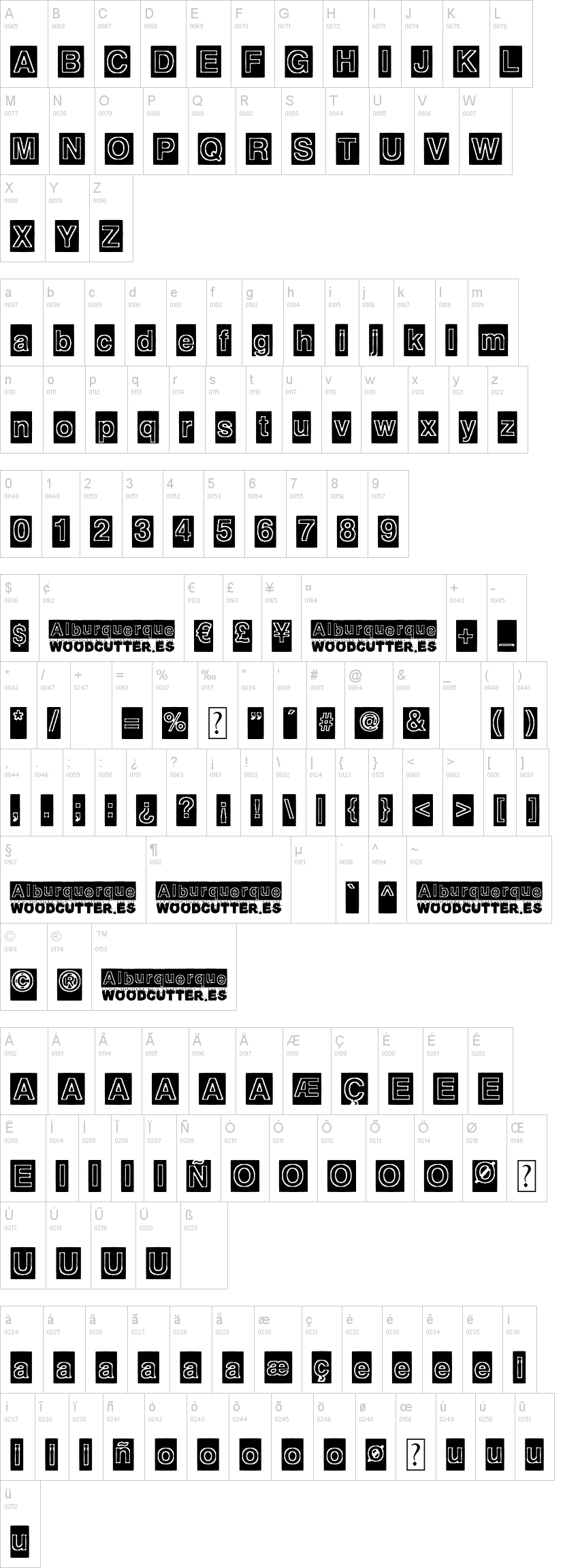The image features a grid of white rectangles outlined in light grey, each containing various elements. The topmost row showcases the alphabet, with each white rectangle featuring a distinct letter prominently displayed at the top. Inside the white rectangles, smaller black rectangles contain white-outlined letters or patterns that are difficult to decipher due to their small size. Below the alphabet row is a section of rectangles filled with more complex patterns and indistinguishable white-outlined letters.

Further down the image, there are longer white rectangles that contain larger black rectangles with grey text inside, followed by clearly legible black text beneath these grey text areas. This pattern repeats multiple times as you move down the image, interspersed with more small black rectangles featuring white outlines of letters or other symbols.

In the lower half of the image, the layout introduces three longer white rectangles with black rectangles and accompanying black text underneath, followed by a row consisting of two smaller black rectangles and one longer one with black text underneath. The final section includes a mix of white rectangles featuring the alphabet letters again, possibly followed by lowercase letters, though these are very small and hard to distinguish.